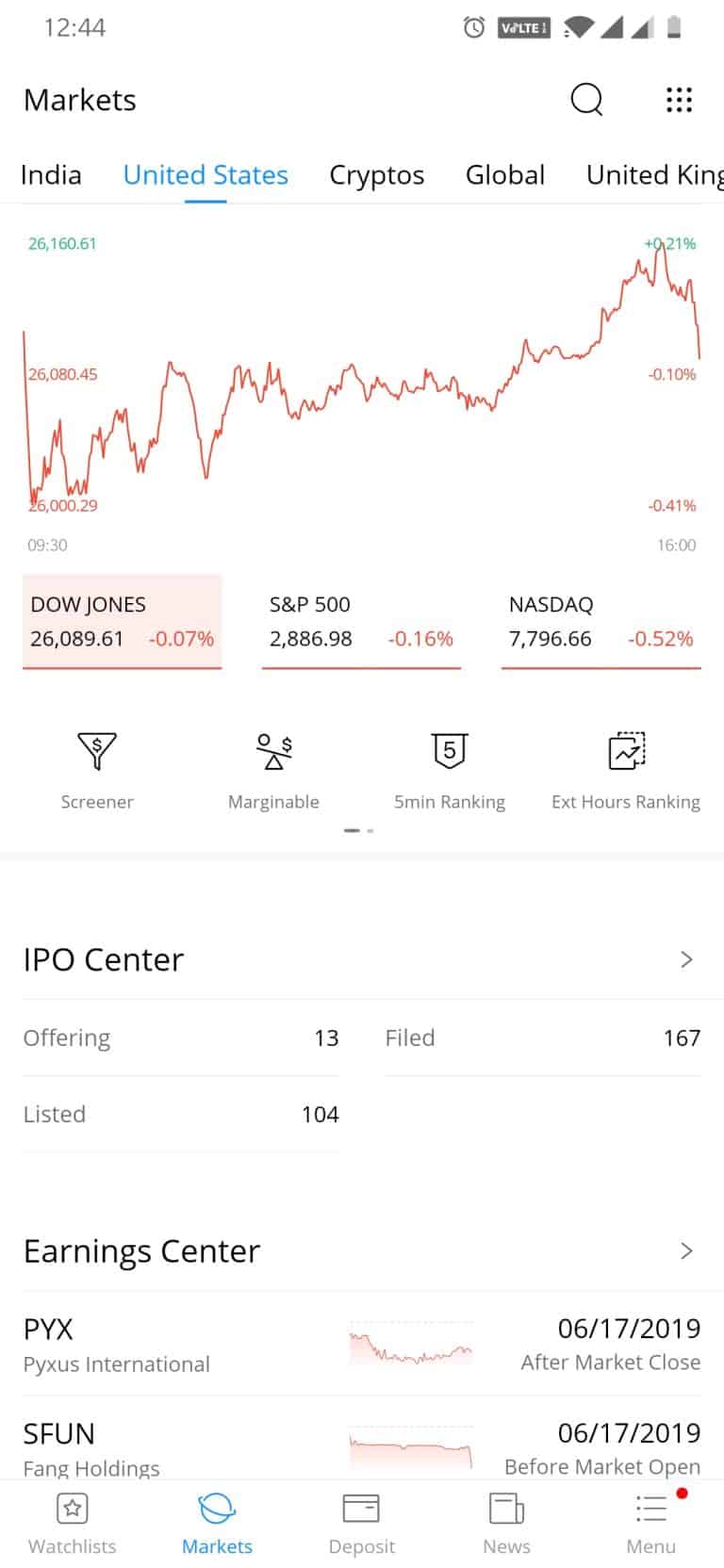In this screenshot of a mobile device, the top bar displays various status icons. At the top left, the time reads 12:44. On the top right, there are multiple icons: an active alarm icon, a "Voice of IOT" icon, a Wi-Fi signal icon indicating full signal strength, a SIM1 icon showing full signal strength, a SIM2 network bar indicating about 70% signal strength, and a battery icon indicating low battery.

Below the status bar, there are several text labels: "Markets," "India," "United States," "Cryptos," "Global," and "United Kingdom."

The image also includes a trading board displaying the current figures for major market indices:
- Dow Jones: 26,089.61, down by 0.07%
- S&P 500: 2,886.98, down by 0.16%
- NASDAQ: 7,796.66, down by 0.52%